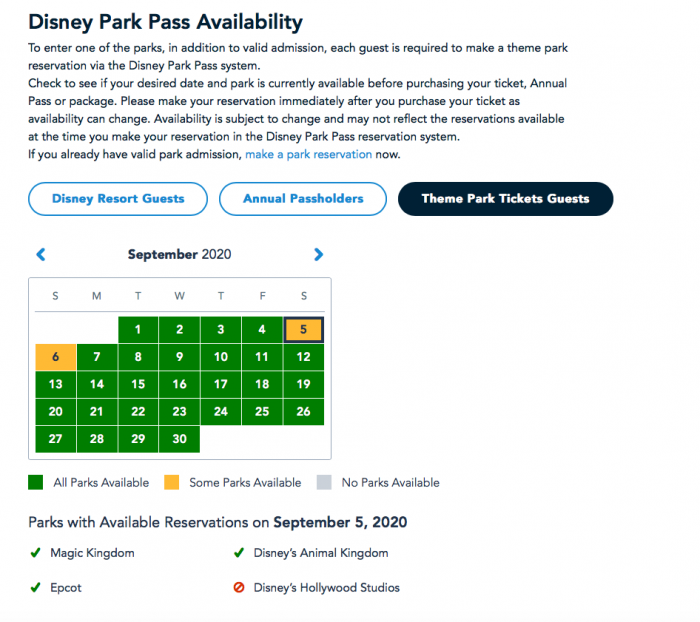This is a detailed screenshot of an informational webpage designed to guide visitors through the Disney Park Pass reservation process. Set against a clean, white background, the page features prominent black text at the top left that reads "Disney Park Pass Availability" in bold font. Positioned just below this heading is a paragraph in smaller, left-justified black text, which provides essential instructions: 

To enter one of the parks, in addition to valid admission, each guest is required to make a theme park reservation via the Disney Park Pass system. Check to see if your desired date and park is currently available before purchasing your ticket, annual pass, or package. Please make your reservation immediately after you purchase your ticket as availability can change. Availability is subject to change and may not reflect the reservations available at the time you make your reservation in the Disney Park Pass reservation system. If you already have valid park admission,

Within this paragraph, the phrase "make a park reservation" is highlighted in blue, emphasizing the action guests need to take immediately. This is followed by a "Now" in black, underlining the urgency.

Below the paragraph, there are three interactive buttons arranged horizontally. The first two buttons are white with medium blue outlines and blue text in the center. They are labeled "Disney Resort Guests" and "Annual Pass Holders," respectively. The third button stands out with its black background and white text, labeled "Theme Park Tickets Guests."

To the left of these buttons is a monthly calendar area. At the top center of this section, the title in bold reads "September," followed by "2020" in regular font. Blue navigation arrows are situated at the far left and right, enabling users to toggle between months. The calendar itself is neatly outlined in thin light gray, featuring a white background. Across the top row are light gray, all-caps letters indicating the days of the week: "S M T W T F S."